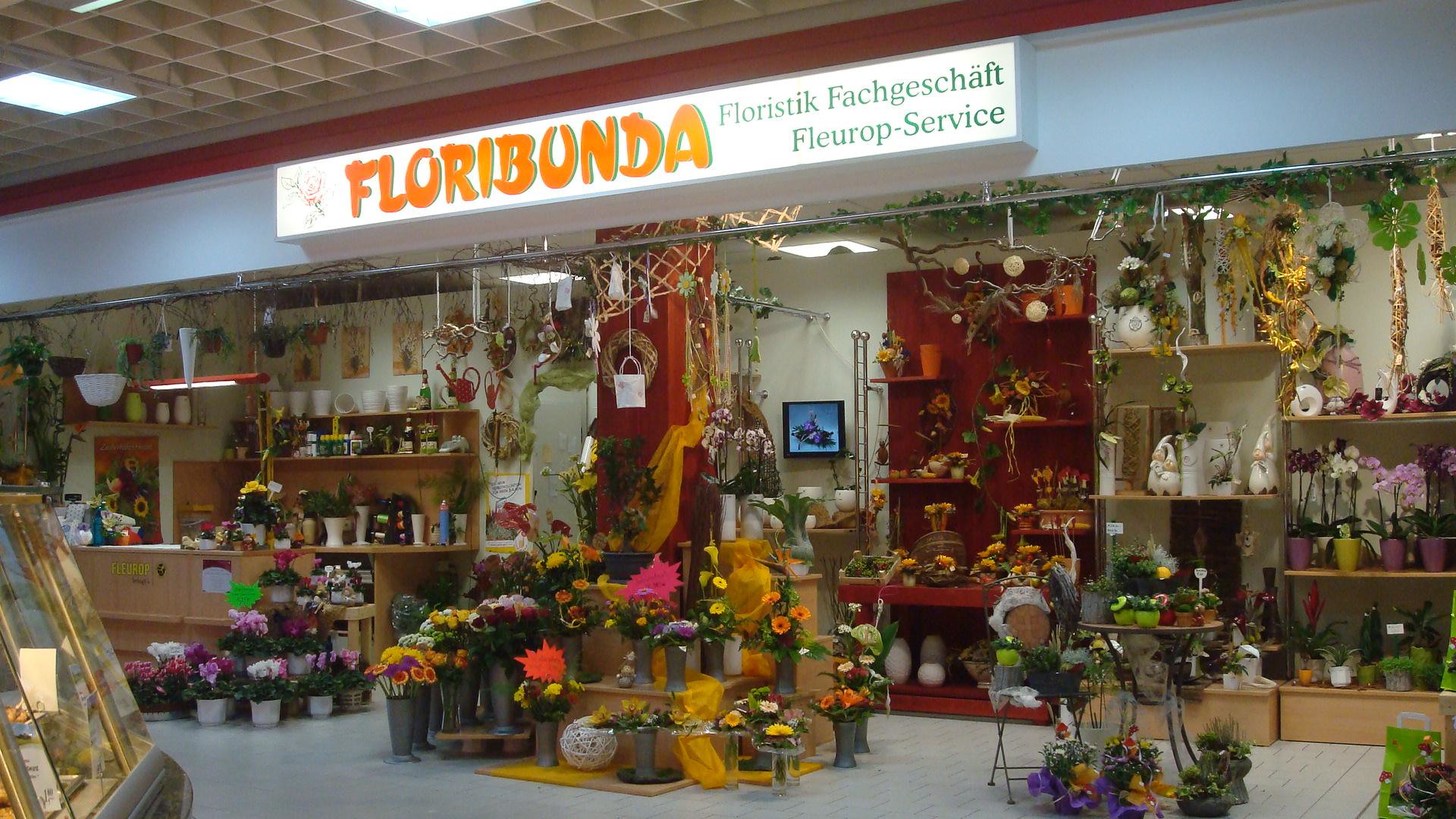This photo captures the vibrant and colorful interior of a flower shop named Floribunda, located inside a mall. The shop features a distinctive sign at the top of its white wall, displaying "Floribunda" in bright orange letters, followed by "Floristic Fachgeschäft" in green, and "Fleurop-Service" in blue lettering. The ceiling is scalloped with sunlights that brighten the entire store.

The store is filled with an extensive and varied collection of flowers and plants. Against the walls, on the shelves, on the ground, and even in the center displays, one can see a diverse assortment of flowers in vivid colors such as orange, pink, burgundy, yellow, white, and purple. Orchids and plain greenery add to the variety. Empty vases, watering cans, and other flower-related items are organized on light brown wooden shelves. The floor in front of the wall is gray, while the overall floor of the store is white, providing a clean backdrop for the colorful displays.

Hanging baskets, pots, and assorted vases filled with flowers contribute to an overflowing appearance, creating a lush and inviting atmosphere. Specially mentioned areas, like the far left background shelving, showcase white vases, bowls, and candlesticks adorned with flowers, adding to the decor. The photo is a detailed, bright depiction of a well-stocked flower shop with flowery displays scattered throughout, emphasizing color and variety.